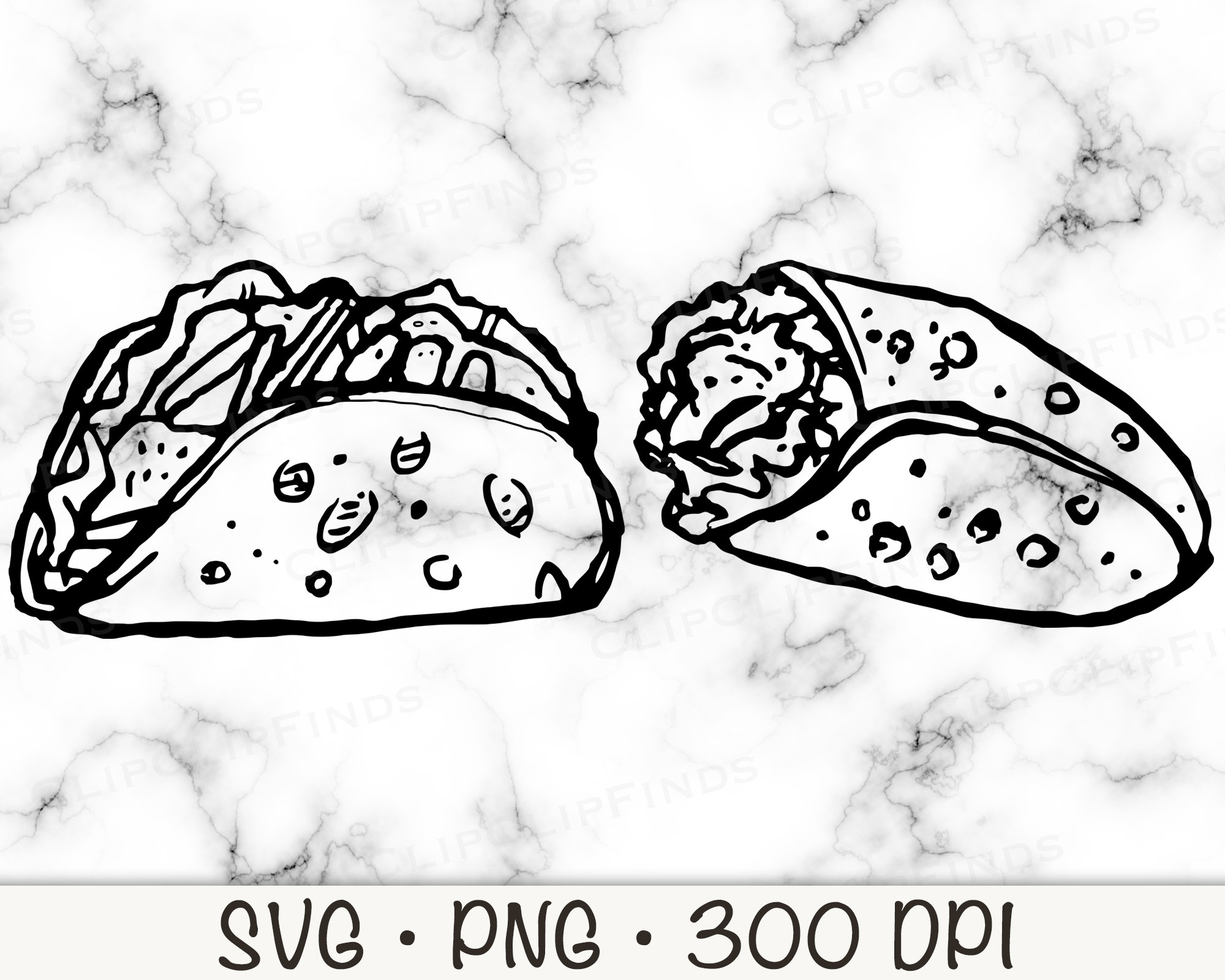The black and white drawing features two distinct silhouettes against a mostly white background with subtle black wisps and squiggly lines creating a marbled effect. On the left side, there is a taco depicted in its characteristic semi-circle shape, filled with various ingredients. To the right, a wrap is depicted, tightly folded to enclose its contents. Both the taco and the wrap are detailed with trademark markings, such as dots and lines, but the exact nature of the ingredients remains indiscernible due to the monochromatic scheme. Beneath these images, in prominent black letters, the text reads "SVG.PNG.300DPI," with gray text and a gray line above it, spanning the width of the drawing. The overall clarity of the image is sharp, making the animated illustrations stand out vividly against the bright and clean background.